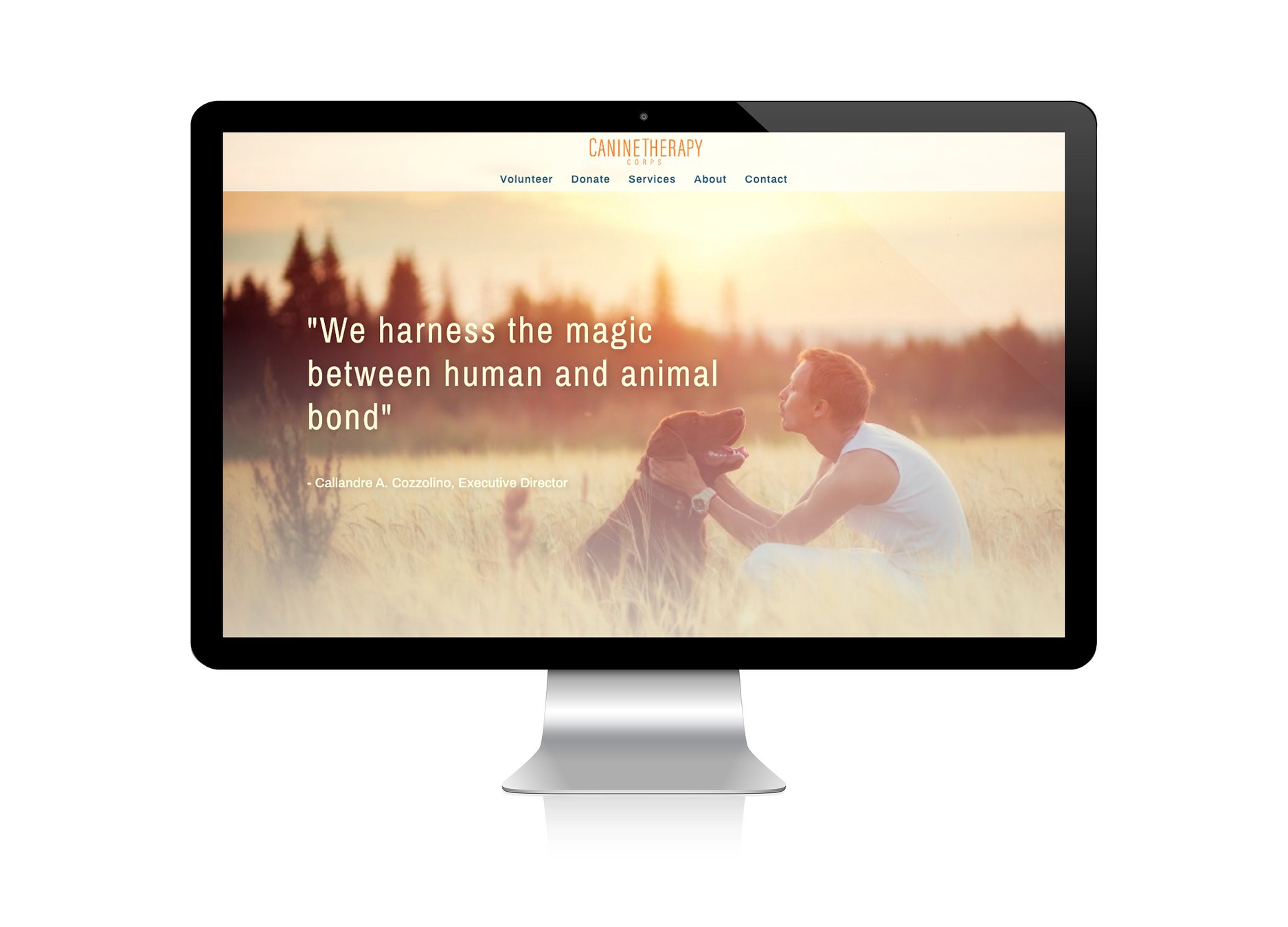The image features a rectangular desktop monitor with a sleek black outline and a silver stand. Displayed on the monitor is a website dedicated to canine therapy. At the top center of the website, bold orange letters spell out "Canine Therapy." Below this heading, text is present but unreadable due to its small size. 

Continuing down the monitor screen, starting from the middle left, the navigation menu includes the word "Volunteer" in plain black text. To the right, subsequent menu items "Donate," "Services," "About," and "Contact" are listed in bold black letters.

Beneath the navigation menu, a captivating photograph captures an outdoor scene in a grassy field, possibly a hay field. The background of the image is artistically blurred, revealing glimpses of trees, a blue sky, and scattered clouds. In the foreground stands a black Labrador dog facing a man who is bent down, tenderly holding the dog’s face with both hands. The man, who has pale skin and short brown hair, is dressed in a white outfit.

To the left of the photograph, an inspiring quote in bold white letters reads, "We harness the magic between human and animal bond." Below the quote, in smaller white text, the caption credits Calendry A. Cozzolino, Executive Director.